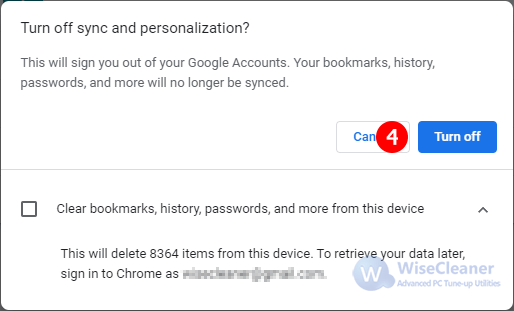**Detailed Caption for the Image:**

The image is a closely zoomed-in snippet of a webpage, focusing on what appears to be a dialog box or a settings menu from a browser. At the top, a white rectangle is connected to another rectangle by a thin gray line, indicating a connection or navigation flow. Each corner of the rectangles (top left, bottom left, top right, and bottom right) features a small dark gray triangle, suggesting a 3D effect or interactive areas to expand the screen.

In bold black text at the top of the image, the question "Turn off sync and personalization?" is displayed. Directly below, in slightly smaller black text, the message clarifies: "This will sign you out of your Gmail accounts. Your bookmarks, history, passwords, and more will no longer be synced."

Adjacent to this message is a cancel button, a rectangle with a gray border and cyan blue text reading "Cancel." Notably, there is a red circle with a white number 4 at the end of this "Cancel" button, possibly indicating an alert or notification related to this action.

To the right of the cancel button, another prominent bold blue rectangle displays the text "Turn off" in bold white font, indicating an option to proceed with turning off the sync and personalization features.

Below these buttons, there's a square with a black border. Within this square, black text reads: "Clear bookmarks, history, passwords, and more from this device," accompanied by an upwards arrow. Additional text explains, "This will delete 8,364 items from this service." It further instructs, "To retrieve your data later, sign in to Chrome as," followed by a blurred-out portion of the user's email address, maintaining privacy.

At the very bottom of the image, a dark gray circle containing a white "W" represents the logo for a presumed business named WiseCleaner. Next to this logo, the text "Advanced PC tune-up utilities" is displayed, indicating the product or service offered.